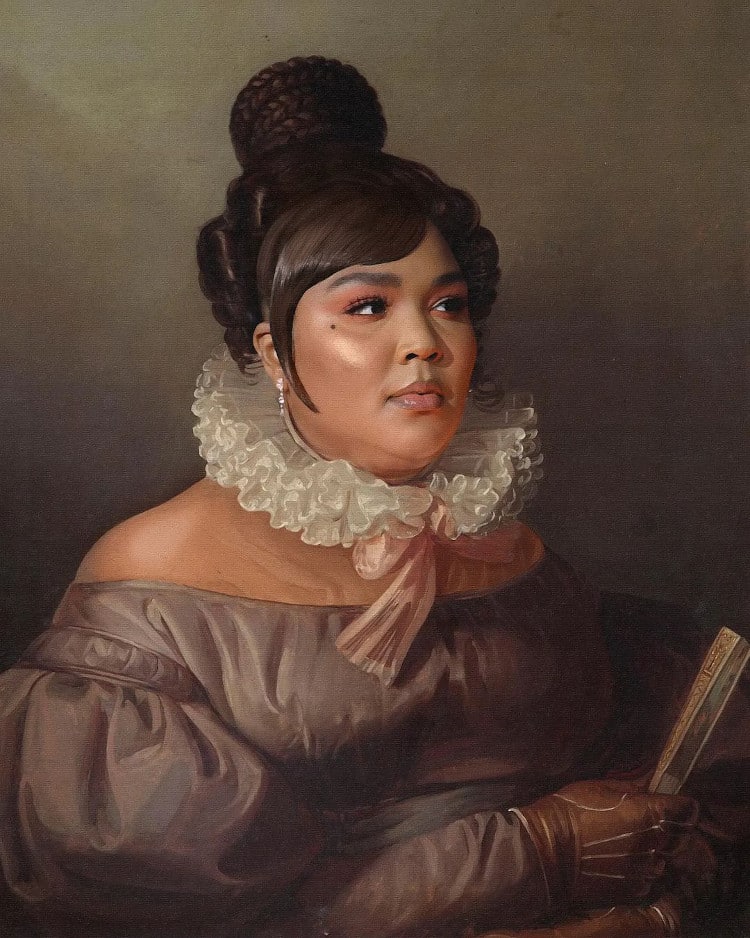The painting features a striking black woman depicted in the style reminiscent of Elizabethan or Victorian portraiture. She has golden-brown skin and is a plus-size model of beauty. Her face, facing towards the right of the frame, is full and adorned with prominent, dark eyebrows and dark eyes, accentuated with makeup. She has full lips with a noticeable cleft below her nose. Her dark brown hair is elaborately styled, with bangs swooped across her forehead and gathered into a tightly woven, curled bun on top, with a few curls cascading at the back.

She is adorned in a light brown or earthy gray off-the-shoulder dress that reveals her elegant shoulders and features puffy sleeves. Around her neck is a distinctive white, ruffled Elizabethan collar with a large pink bow. Her ensemble is complemented by a pair of brown leather gloves. In her right hand, she delicately holds a Japanese-style fan, which is closed. She also wears a single white pearl earring, adding to her refined appearance. The artist employs dark, earthy tones to enhance the painting's timeless and classical aura, blending historical aesthetics with a modern portrayal.